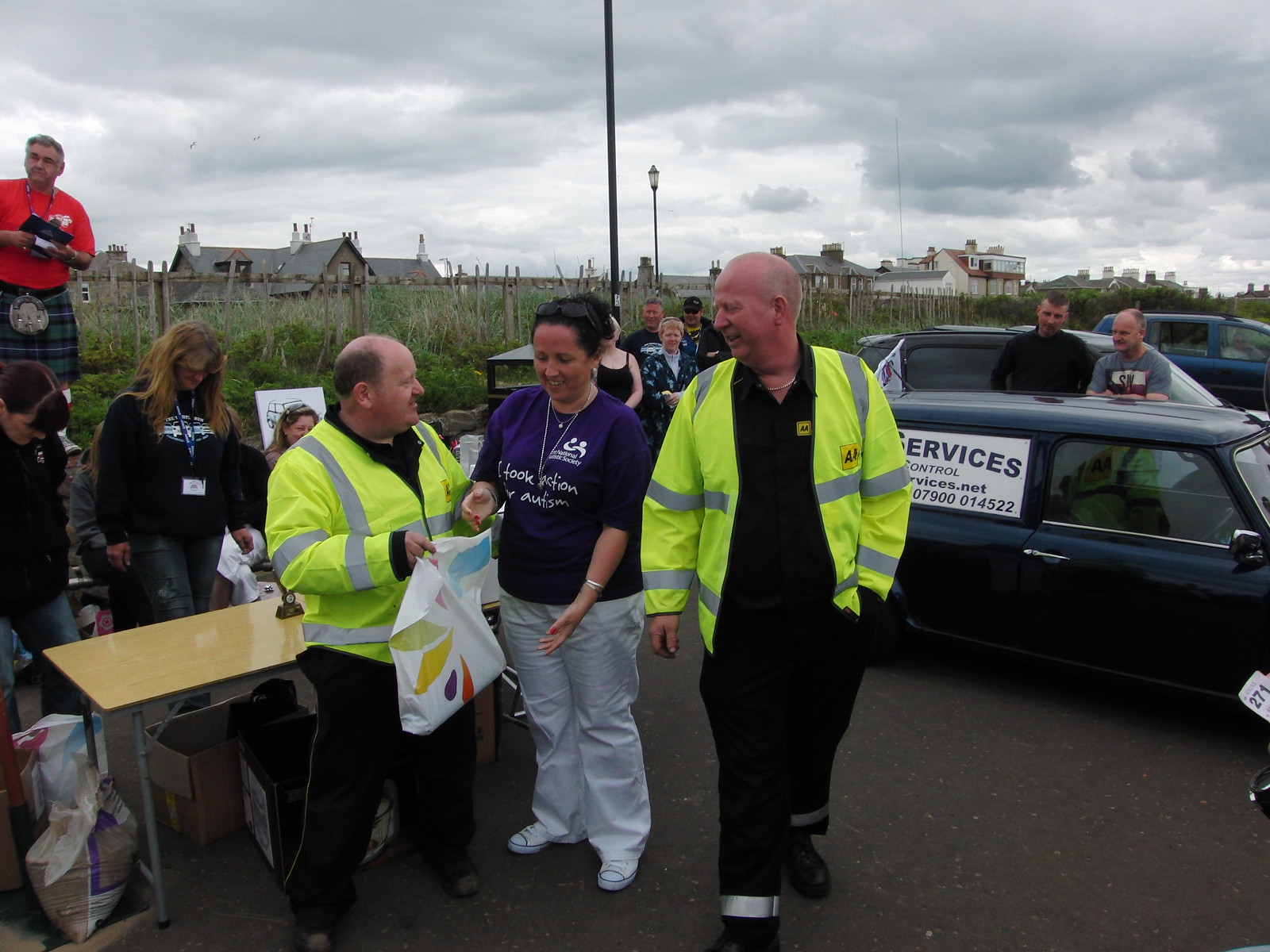In this outdoor photo taken on a gloomy, cloudy day, a group of people is gathered in what appears to be a parking lot or street, possibly for a charity event. Prominently in the center are three individuals: a bald man on the left, sporting a mustache, and dressed in a yellow high-visibility jacket with "AA" in black text, and dark pants. He holds a white plastic bag covered in colorful designs. Next to him, a woman with dark black hair tied in a bun, wearing a blue t-shirt that reads "I took action for Autism," white pants, a necklace, and sunglasses, extends her hands toward the bag. To her right stands another bald man, taller, in a bright fluorescent yellow jacket with another "AA" patch, a black shirt, and pants, looking down toward the shorter man.

Behind them is a small, beige, fold-up wooden table surrounded by people—men and women, some standing, some sitting. In the background, a black car with a white "services" sign is visible, with two men standing behind it. Above them, there are three cars and a wooden fence bordering a grassy slope, which leads to a line of houses. To the top left of the image, a man wears a red shirt and kilt, positioned on a stone wall. The scene is accentuated by tree branches and roofs of buildings, enhancing the setting's dreary atmosphere.